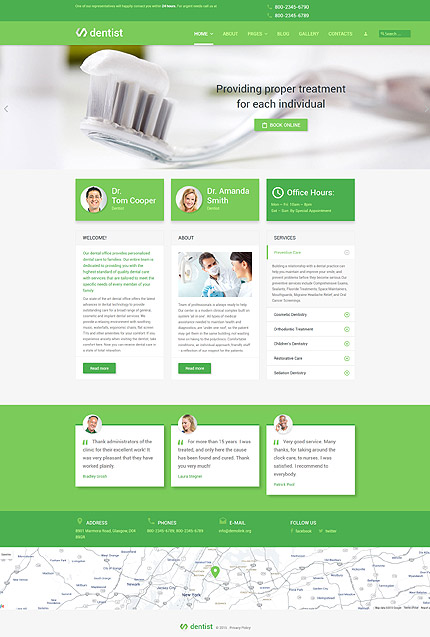This vertically oriented rectangular image showcases a website dedicated to dental services. At the very top, there's a dark green border featuring a tiny white blurb that is difficult to read due to its minuscule size. This border also contains two toll-free phone numbers, suggesting easy contact options. Directly below, a light green border presents a white dental symbol on the left side, adjacent to the word "Dentist" in white text.

Next to this, there's a faintly visible navigation menu listing options: Home, About, Prices, Blog, Gallery, and Contacts, with the 'Home' section currently selected and underlined.

As the eye moves further down, the background displays a close-up image of a toothbrush with toothpaste. To the right of the toothbrush, bold black text reads "Providing Proper Treatment for Each Individual." Below this message, a prominent green button with white text invites visitors to "Book Online."

Further down the page, there are three rectangular boxes aligned horizontally. The first on the left is labeled "Dr. Tom Cooper," the second in the middle reads "Dr. Amanda Smith," and the third on the right provide "Office Hours," which offers crucial information about the availability of the dental services.